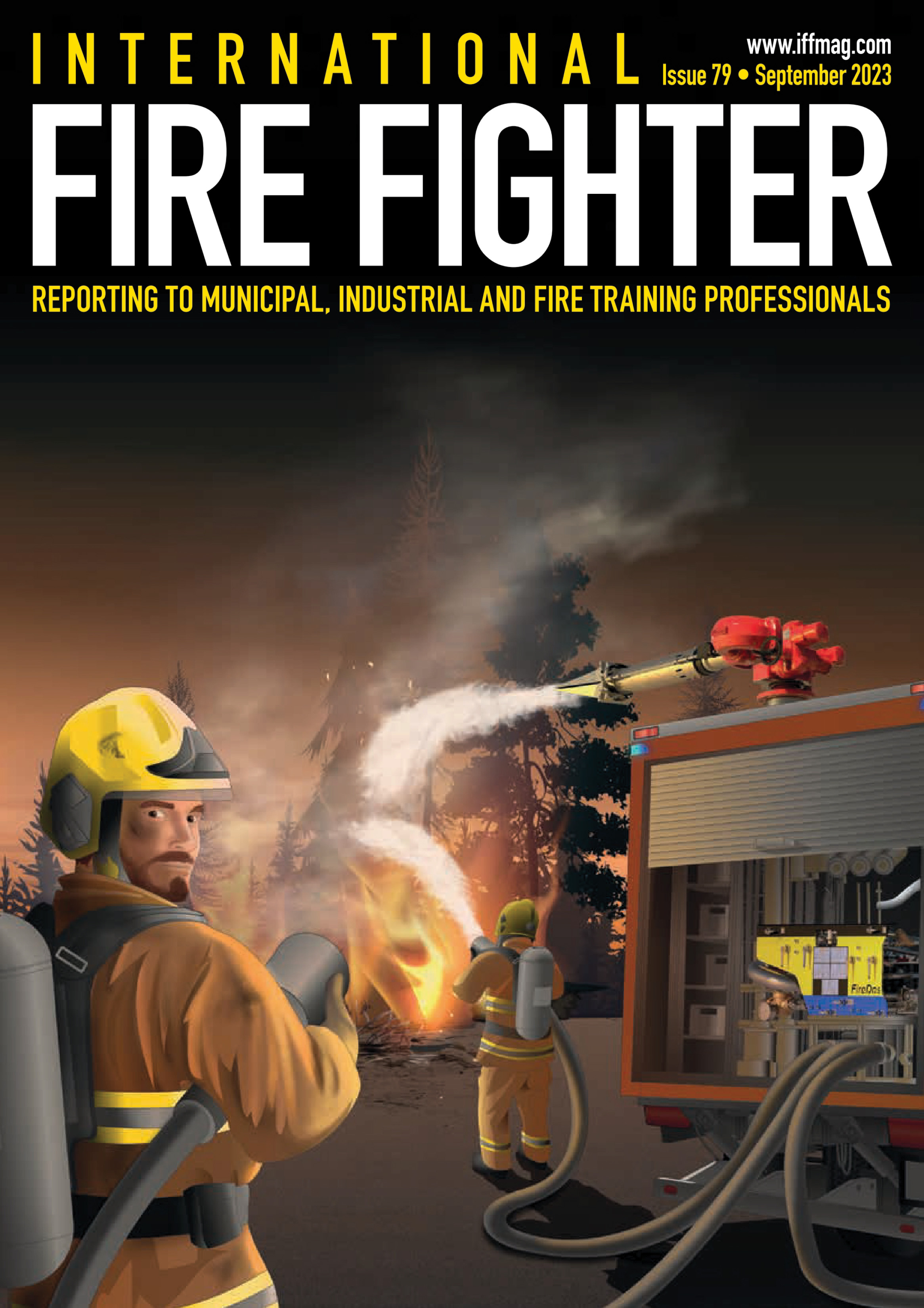The cover of the International Firefighter Magazine, Issue 79, September 2023, features a detailed, computer-generated 3D artistic rendering of firefighters combating a forest fire. The sky in the background is a dramatic mix of black, brown, and orange, emphasizing the severity of the blaze. At the very top of the cover, the title "International Firefighter" is prominently displayed—'International' in yellow letters and 'Firefighter' in bright white. Just beneath the title, in yellow, it states, "Reporting to Municipal, Industrial and Fire Training Professionals," and the web address, www.iffmag.com, is situated in smaller font at the very top.

In the lower left-hand corner of the cover, a firefighter dressed in traditional gear, including a yellow helmet, is holding a hose with his right arm. He is glancing back over his right shoulder, making eye contact with the viewer, his Caucasian face framed by a brown beard and mustache. His dark eyes convey determination. The central part of the image showcases another firefighter mid-action, directing a powerful stream of water at a tree engulfed in flames. To the far right, an opened fire truck can be seen with hoses extending from it, and atop the truck, a mounted nozzle shoots additional water at the blazing trees.

The scene is vivid with contrasting colors—the dark hues of the night sky punctuated by the bright, fiery oranges of the forest fire, complemented by the light browns and yellows of the foreground elements. This dynamic and intense cover compellingly captures the bravery and urgency of firefighting professionals.